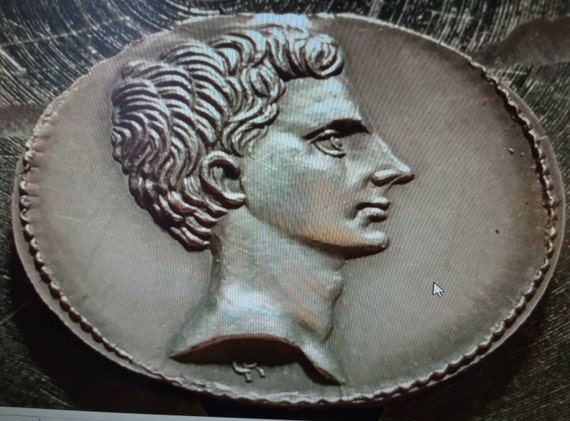The image is a highly detailed, close-up color photograph of an ancient Roman coin, presented in a monochrome style. The square photo depicts this singular coin placed against a dark, brown surface, likely wood. The background features a stark blackness interspersed with white lines, and there is a small gray border visible at the lower left corner. The main subject, the coin, showcases a side profile of a man gazing rightward. His curly, wavy hair, pronounced nose, eyes, and prominent chin are meticulously detailed, contributing to the coin’s worn silver, tarnished texture. The coin's rim displays a rough texture, further enhancing its ancient appearance. The overall clarity of the image is sharp and bright, due to ample natural lighting.